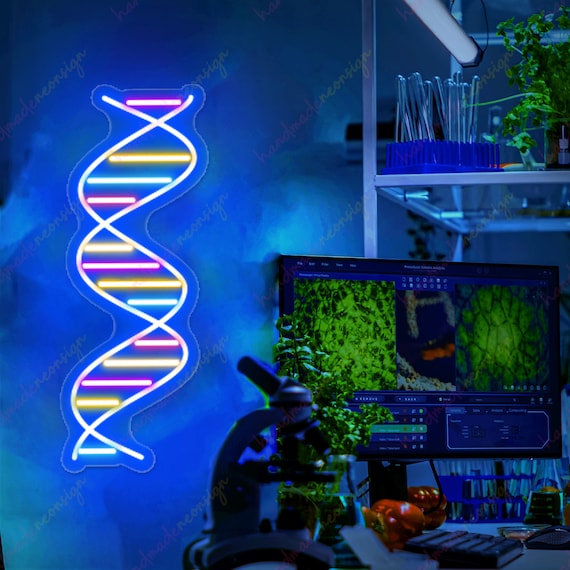In this square nighttime indoor photograph, the focus is drawn to a meticulously arranged desk situated in the lower right corner. The blue wall on the left is adorned with a neon light, featuring three squiggly lines that form teardrop shapes, illuminated in white, yellow, blue, and pink horizontal neon strips. Dominating the desk is a large screen monitor positioned toward the left side. Adjacent to the monitor on its left is a sleek black microscope, hinting at scientific explorations. Beneath the monitor are two mysterious red objects that resemble apples in shape, adding a splash of color and curiosity. The background of the desk reveals stacks of what appear to be CDs, adding a nostalgic touch to the modern setup. The contrasting elements of vibrant neon art and technological instruments create a captivating and visually stimulating scene.